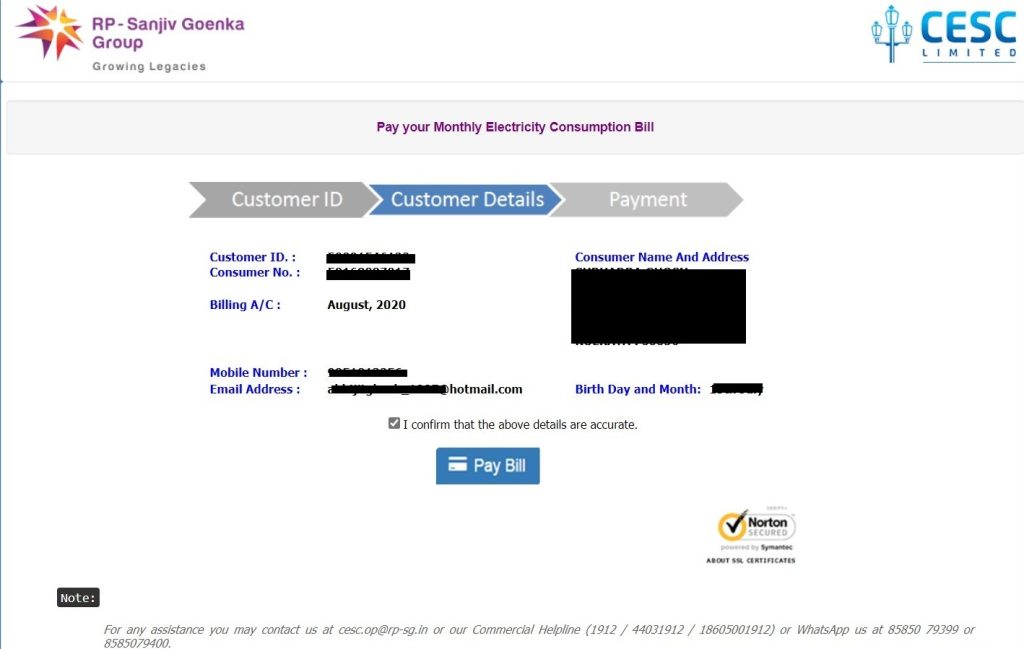"This image depicts an electric bill issued by CESC Limited, a part of the RP Sanjiv Goenka Group. The top left corner features 'RP Sanjiv Goenka Group' written in purple letters, with 'Growing Legacies' in black letters beneath it. Next to this text is a distinctive logo in purple and orange that almost forms a star. On the right-hand side, 'CESC Limited' is prominently displayed in blue capital letters alongside a blue illustration of a light pole. Beneath this, 'Pay Your Monthly Electricity Consumption Bill' is written in purple letters.

The bill contains sections labeled Customer ID, Customer Details, and Payment. Key details like the Customer ID, Consumer Number, mobile number, email address, Consumer Name, and Address are blacked out for privacy. The billing period is specified as August 2020. There is a section to confirm the accuracy of the details, which is checked.

A blue button labeled 'Pay Bill' in white letters is present, accompanied by a small blue and white credit card icon. The bill indicates it is protected by Norton Antivirus, evident from the icon displayed on the document.

At the bottom, a note provides contact information for assistance, including an email address (CESC.OP@rpsgin.in), a commercial helpline phone number, and a WhatsApp number for support."